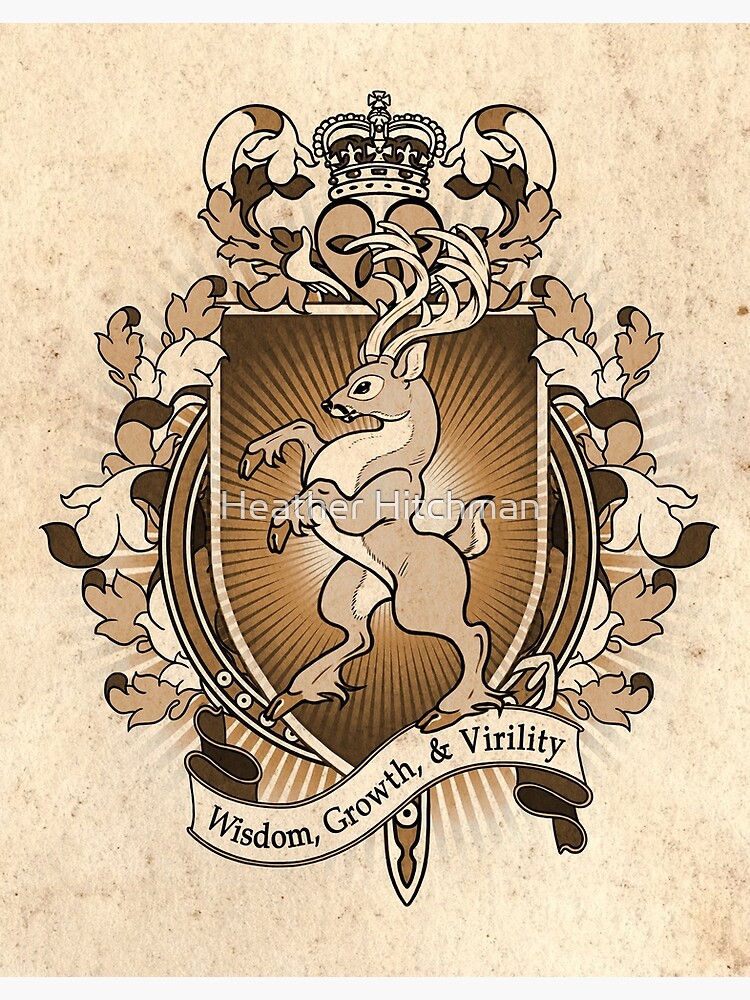The image depicts a family crest with a detailed shield as its centerpiece. The shield, colored in shades of brown and tan, features a flat top, curved sides, and a pointed bottom, reminiscent of a sunburst design. In the center of the shield stands a light brown deer on its hind legs, poised as if ready to box, with large, white antlers facing left. The deer has a white belly, adding to its distinct appearance. Above the deer is a decorative heart crowned with a regal crown. Surrounding the shield are intricate, wavy leaf-like designs in varying shades of brown and white. Below, a light-colored, curved banner bears the words "wisdom, growth, and virility" in black text. The entire crest is set against a stone beige background speckled with dark spots, and the name "Heather Hitchman" is written in white at the top.